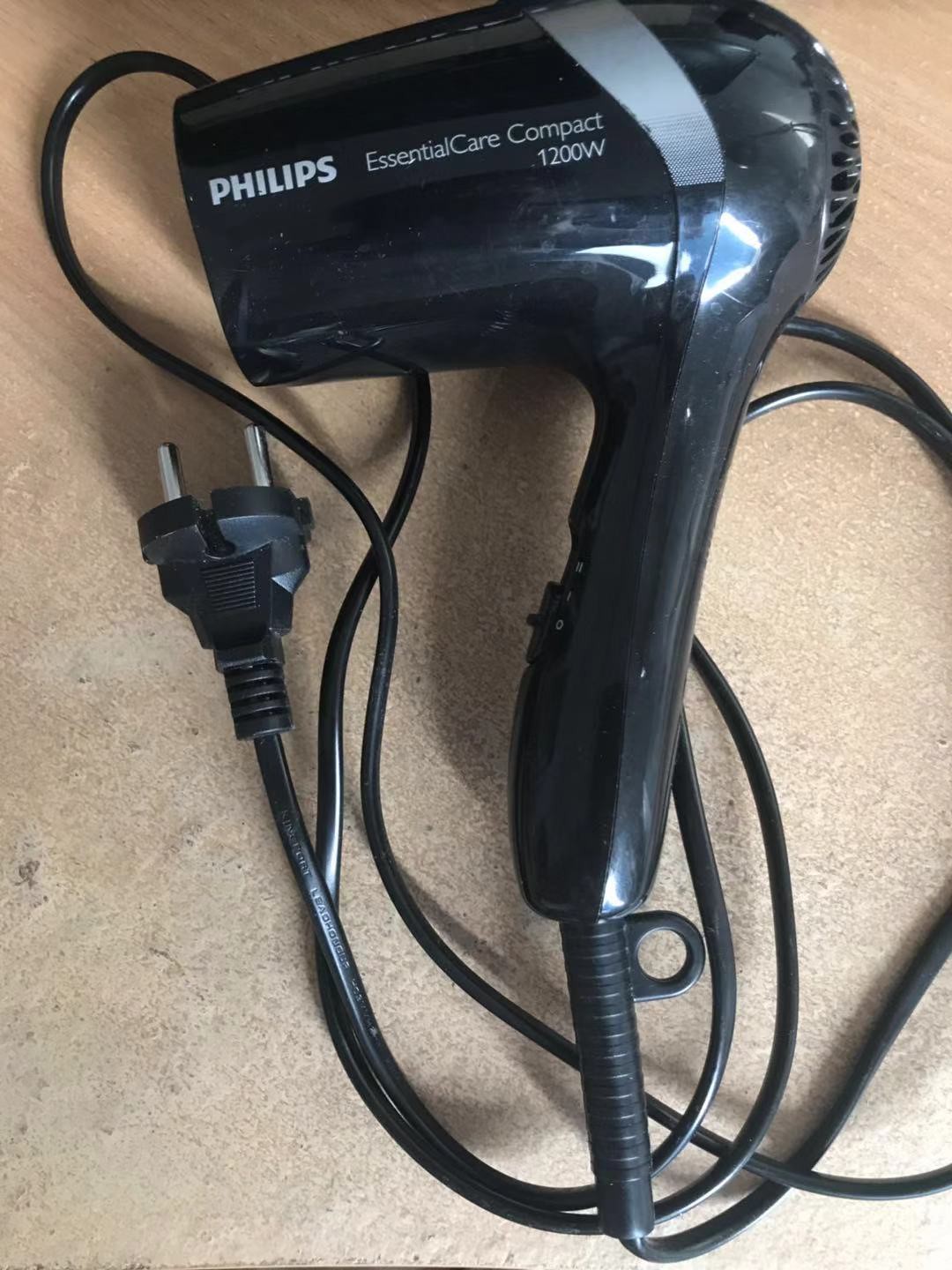This detailed photograph showcases a compact, black Philips Essential Care hairdryer (1200W), prominently positioned in an up-close view that makes the appliance appear larger than its actual size. The branding "PHILIPS Essential Care Compact 1200W" is clearly displayed in white lettering, just above a silver stripe located near the air intake at the top. The black handle and vented exhaust fan are also visible. The hairdryer is unplugged and rests on a tangle of its own electrical cord, which features a standard AC adapter plug. The scene is set on a jagged, wooden surface, likely a table or shelf, with a brightly lit background that casts distinct shadows of both the hairdryer and the plug.